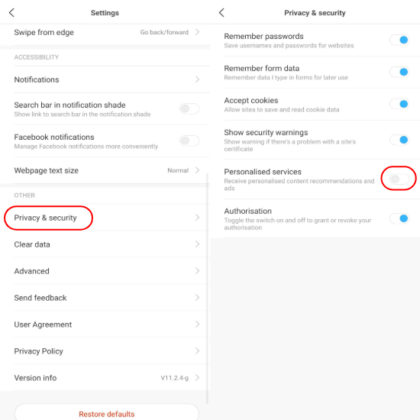This detailed screenshot captures the "Settings" page, focusing on "Privacy and Security" options on an Android device. The image highlights specific elements with digitally-added red circles, emphasizing key sections like "Privacy and Security" and "Personalised Services," the latter of which is turned off. Other notable settings that are enabled include "Remember Passwords," "Remember Form Data," "Accept Cookies," "Show Security Warnings," and "Authorization." The "Restore Defaults" option is prominently displayed at the bottom in red font. For clarity, the version information is listed as 11.2.4g, designated for illustrative purposes.